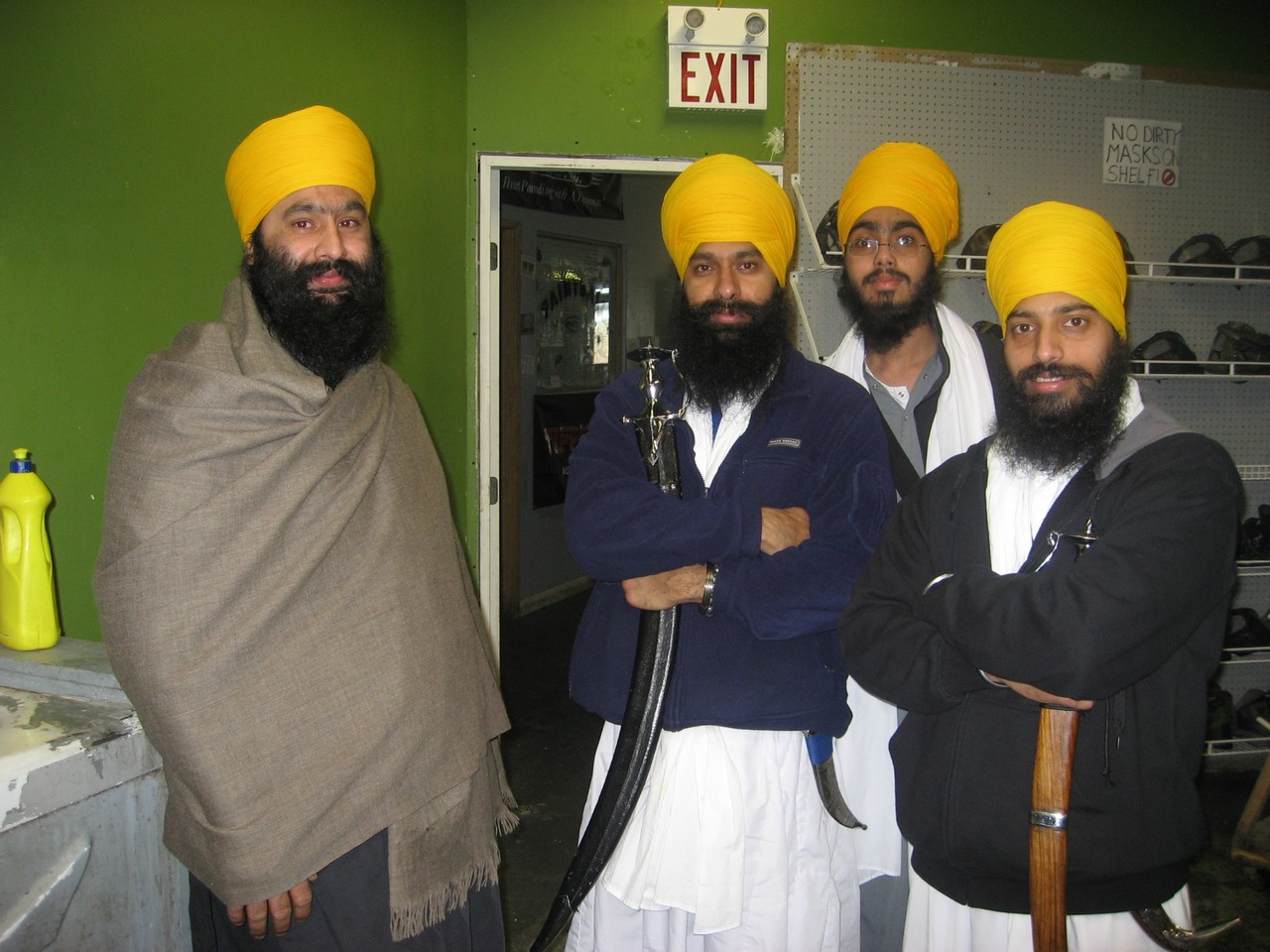The photograph captures a group of four Indian men, each adorned with yellow turbans and sporting long black beards and mustaches. They stand in what appears to be a room with green walls, partially painted in a green hue, featuring white shelves attached to one wall and a gray section with racks that hold hats. The backdrop includes an open door marked with a red exit sign, revealing some equipment, possibly a washing machine and a yellow bottle. 

From left to right, the first man is draped in a shawl covering his entire upper body. The second man dons a blue sweater over traditional white robes and holds a long curved scimitar. The third man wears a black jacket over his white robes, while the fourth man, also in a black jacket over white robes, carries a scimitar with a brown sheath. Two of the men, positioned in the front, have their arms folded across their chests. All four men wear traditional white tunics and pants, combined with modern jackets, creating a blend of traditional and contemporary attire. The scene suggests a posed photograph, likely taken in a business setting.